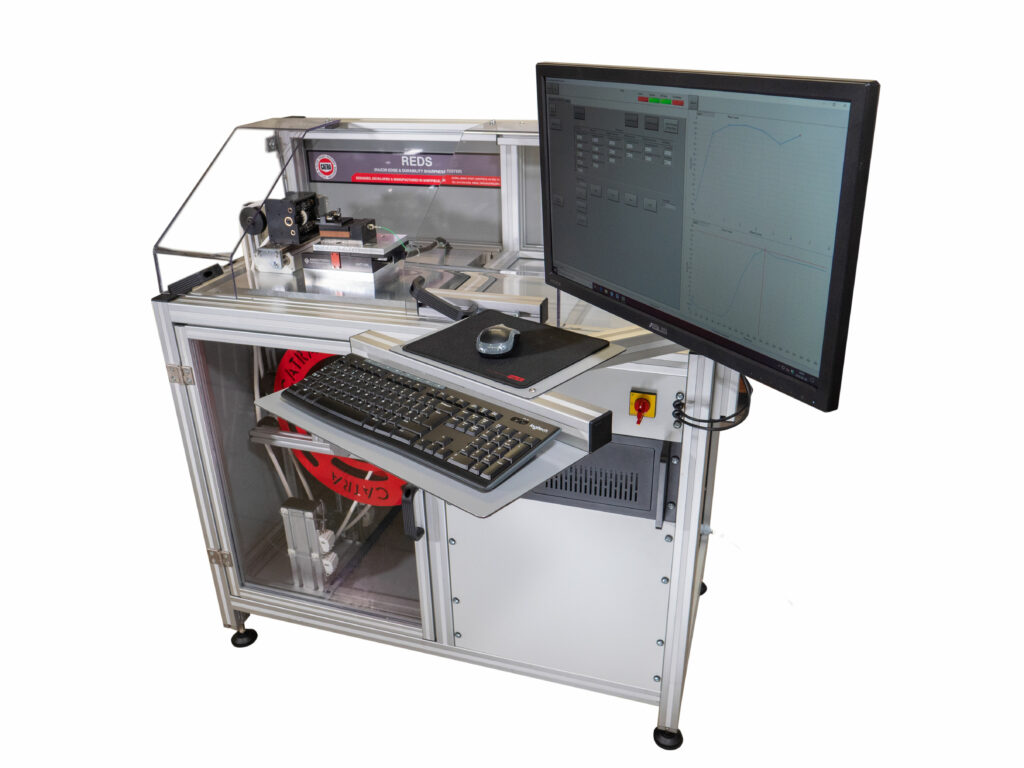This is a detailed photograph of a sophisticated machine setup, possibly a milling machine or a 3D printer, housed within a large, metallic, rectangular cabinet with four black-tipped feet for support. The cabinet features two distinct sections: the left side with a glass door, through which a red wheel and some machinery are visible, and the right side with a gray grill. Despite no people or animals being present in this color photograph, there is considerable focus on the machine’s operation.

On top of the silver cabinet, enclosed in a glass case, is the machine itself, which has a silver base, a black top, and a black box on its right side, with another black wheel located at the top left. Additionally, a computer console is attached to the machine, including a monitor tilted to the right, mounted on one of the cabinet's protruding poles. The monitor displays a graph and some illegible text. Below the monitor, a tray swings out to support a keyboard and mouse on a black mouse pad. At the back of the monitor, a label reads "R-E-D-S." The entire setup, complete with mechanical parts beneath the cabinet table and visible machinery through the glass, suggests a highly functional and integrated technical work unit.